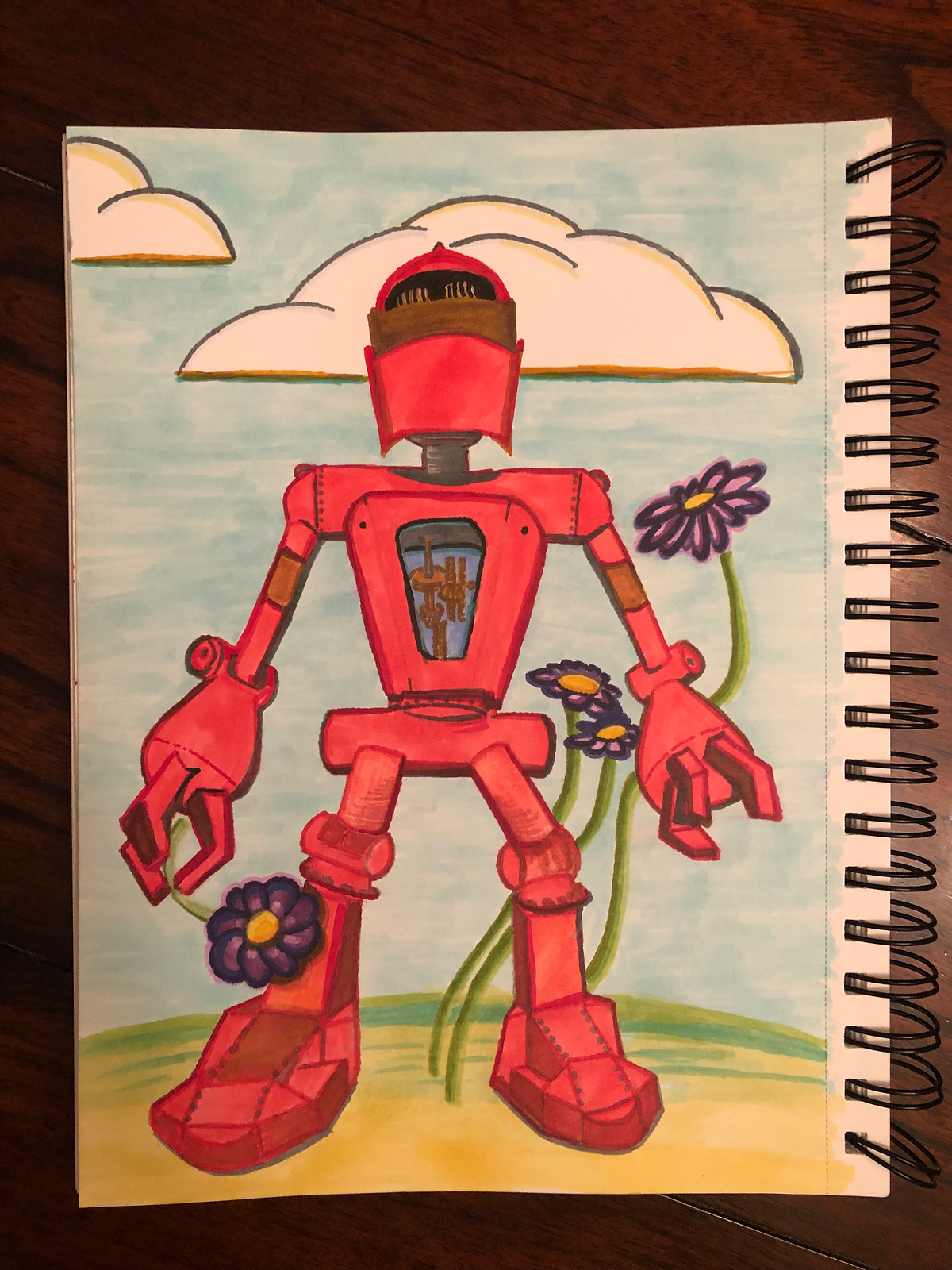In this high-resolution, color illustration, we see a meticulously detailed sketch of a red robot depicted on a page from a spiral-bound notepad folded onto one side. The notepad, held together by double black metal bindings with two rings per square hole along the right side, has a perforation indicating the page can be torn off. The background features a richly dark-stained wooden surface, setting a rustic tone.

The red robot, central to the composition, has a squared-off jawline and a black visor covering its eyes, contributing to its medieval helmet-like appearance. Its chest is illustrated as an inverted triangle, transparent enough to reveal intricate inner gears, emphasizing its mechanical nature. The robot’s arms, slender and metallic, end in three-fingered claws. Its legs lead down to broad feet, suggesting stability.

In its right hand, the robot delicately holds a purple flower. The scene is set against a yellow-green landscape with brown ground featuring tufts of grass. Additional purple flowers rise from the ground, towering beside the robot, complementing the serene, clear blue skies that are dotted with a few fluffy clouds, adding a dreamy and picturesque backdrop to the otherwise mechanical protagonist.